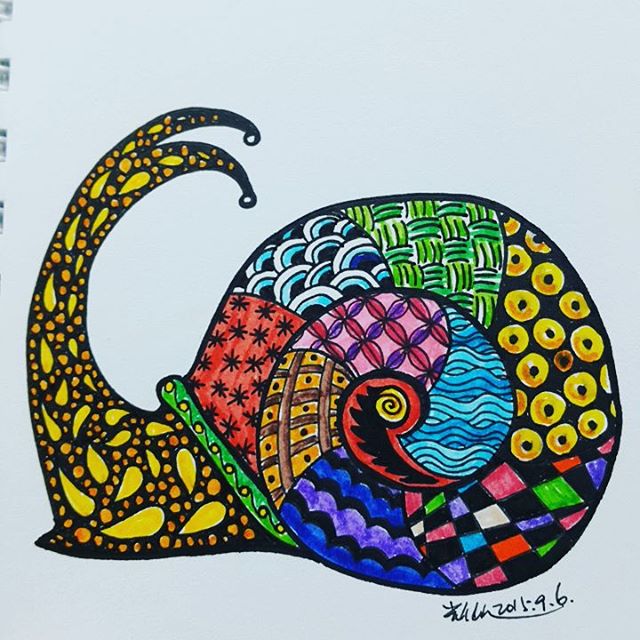In this rectangular image, which is oriented horizontally, we see a beautifully colorful and artistically drawn picture of a snail. The artwork features intricate multi-patterns within the outline of the snail, resembling a creation made with markers. The snail's shell is depicted as curled inward, and two tentacle-like appendages arch back from its head over the top of the shell. The image is rich in a variety of vibrant colors, including blues, reds, yellows, black, green, orange, brown, purple, and pink.

The composition places the snail with its shell facing east and its head facing west. Below this artistic rendering, there is a scribbled signature in what appears to be a thin black marker, though it is not legible. However, the date included is clear, reading "2011-9-6."